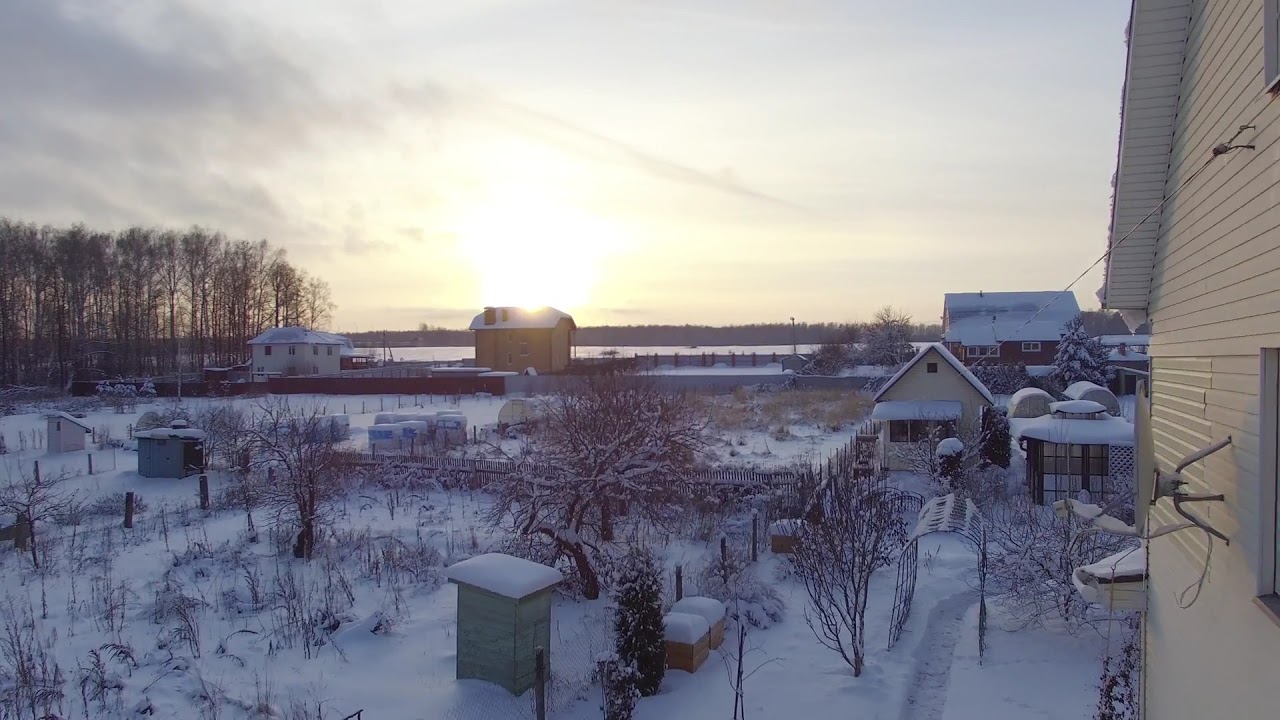The full-color photograph, captured either right after sunrise or just before sunset, depicts a tranquil winter scene in a residential area, outdoors during the daytime. The horizontally rectangular image is borderless, showing a mostly clear sky with some clouds in the upper left-hand corner. Several bare-limbed trees punctuate the landscape. The ground, as well as the roofs of the homes, is blanketed with snow.

The image contains multiple homes, including yellow and red ones, and several smaller buildings. A notable feature is a satellite dish protruding from one of the homes. There is no text visible anywhere in the image. A narrow plowed path, serving as a walkway, meanders through the snow, passing under a decorative garden arch. Scattered around, various plants poke through the snow's surface. The scene's colors include white, brown, green, orange, yellow, tan, and black, arranged in a seemingly random yet harmonious fashion. No people are visible in the serene, snowy setting.